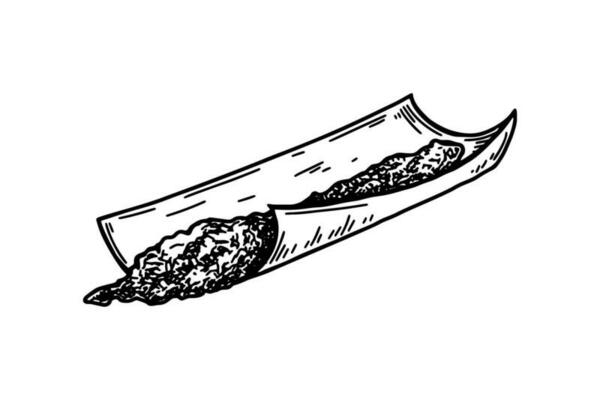This black and white image features a small piece of paper with its edges rolled, indicative of an attempt to construct a handmade cigarette. The paper is irregularly shaped, with a thicker accumulation of what appears to be tobacco concentrated at one end, tapering off towards the other. The uneven distribution suggests an initial attempt to arrange the tobacco within the paper, though it has yet to be properly rolled into a uniform shape. The white background of the photo accentuates the details of the curling paper and the texture of the tobacco, capturing a moment in the process of crafting a cigarette by hand.